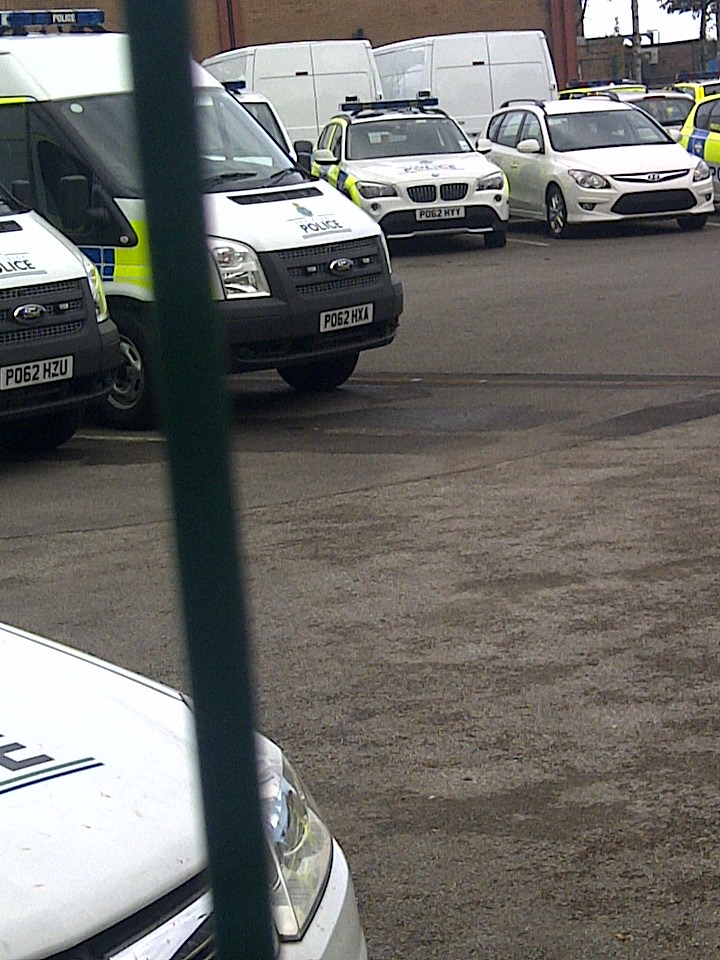The image depicts a parking lot with an array of police vehicles against a backdrop of light and dark brown buildings. The ground is a dark blackish asphalt. On the left side of the image, there are multiple white police vans adorned with blue font reading "police" and yellow markings. These vans have license plates visible on the front, including one with the number 62HZU. In front of these vans, there is a pole running vertically through the image. Toward the center, there's a police car featuring yellow and blue stripes on its side. On the far right, a white Hyundai is parked. The police vehicles, both cars and vans, have distinguishing features such as blue lights on top and the word "police" displayed on the front hoods, with some vans also bearing the Ford logo on a black grille.